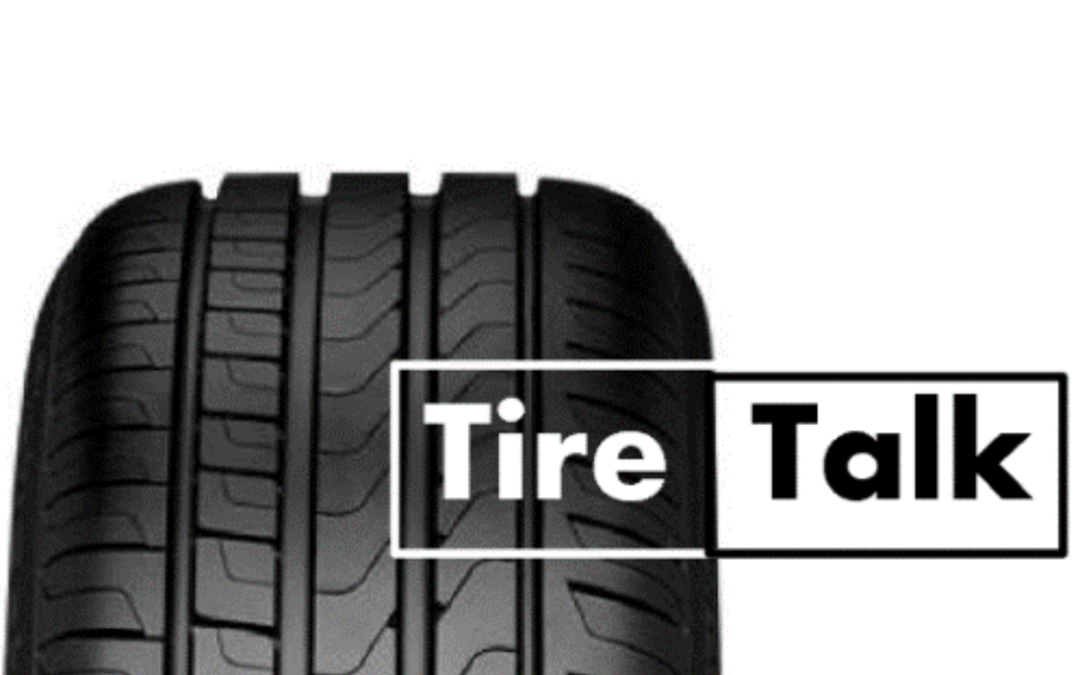The image appears to be an advertisement, possibly for a podcast or a video series about tires. Set against a white backdrop, it features a black tire positioned on the left side, showcasing detailed, fresh treads with both straight and curved grooves to enhance traction. Superimposed over the left side of the tire is a white rectangle with the text "Tire" in bold white font, with the first letter capitalized and the rest in lowercase. Adjacent to this, extending to the right of the tire, is a black rectangle containing the word "Talk," also in bold font with a capitalized "T" and lowercase "alk." Together, these elements form the phrase "Tire Talk," with a clear distinction between the white and black sections of the rectangle. The overall impression is that of a polished, possibly AI-generated or computer-generated image, suited for a promotional context.